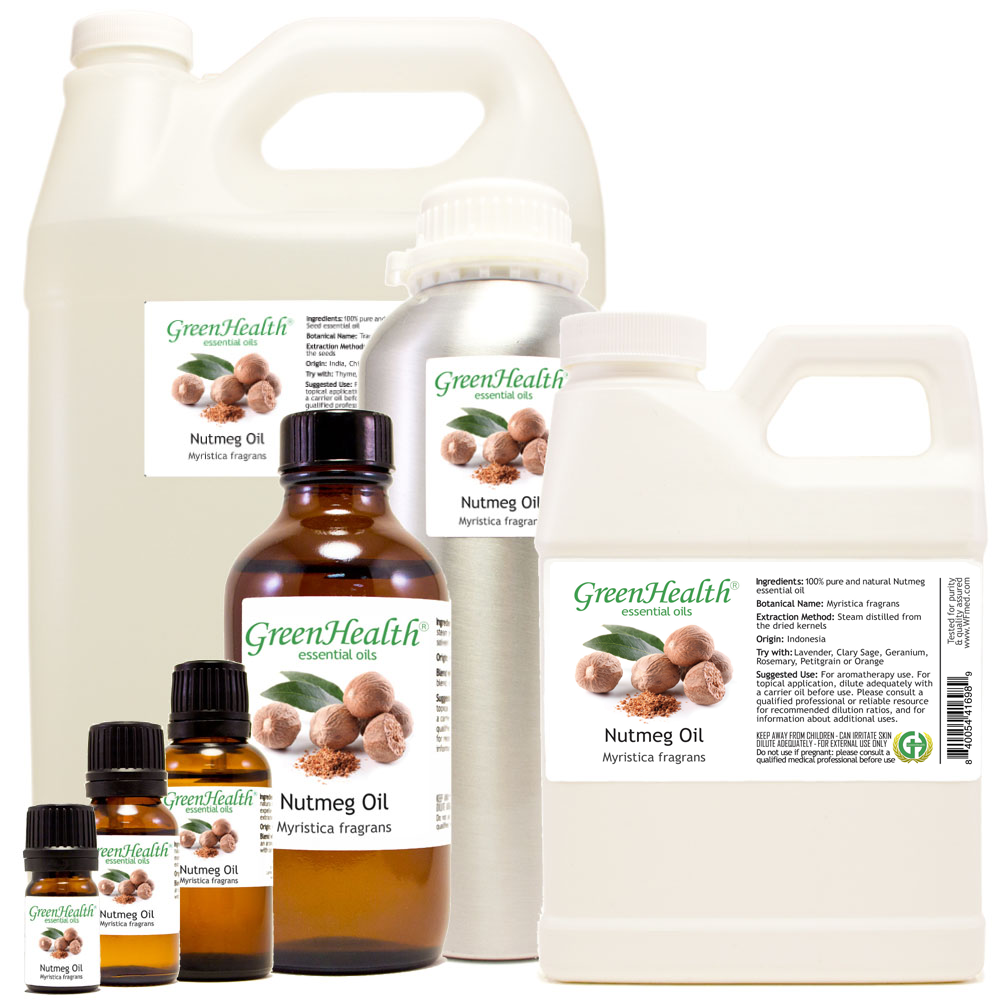The image appears to be an advertisement for Green Health Nutmeg Oil, showcasing the variety of container sizes available for purchase. The background is plain white, allowing the focus to be solely on the product lineup. Central to the arrangement, there is a large white plastic jug labeled "Green Health Nutmeg Oil," featuring images of ground nutmeg, whole nuts, and green leaves. Positioned in front of this jug is a metal canister resembling a thermos, also branded with the Green Health Nutmeg Oil label, specifically highlighting "Myristica Fragrance." 

Adjacent to the thermos-like container is a smaller white jug prominently displaying details such as "100% Pure and Natural Nutmeg Essential Oil," the botanical name, extraction method, origin, and suggested use. Completing the display are four amber glass bottles with black lids, arranged in ascending size order from smallest to largest, each bearing the same Green Health Nutmeg Oil label. These bottles emphasize the gradient of sizes available, starting from tiny dropper bottles to a size comparably several gallons. The cohesive labels across all containers include essential information like ingredients, usage instructions, and a barcode, emphasizing the comprehensive branding and professional presentation of the product line.